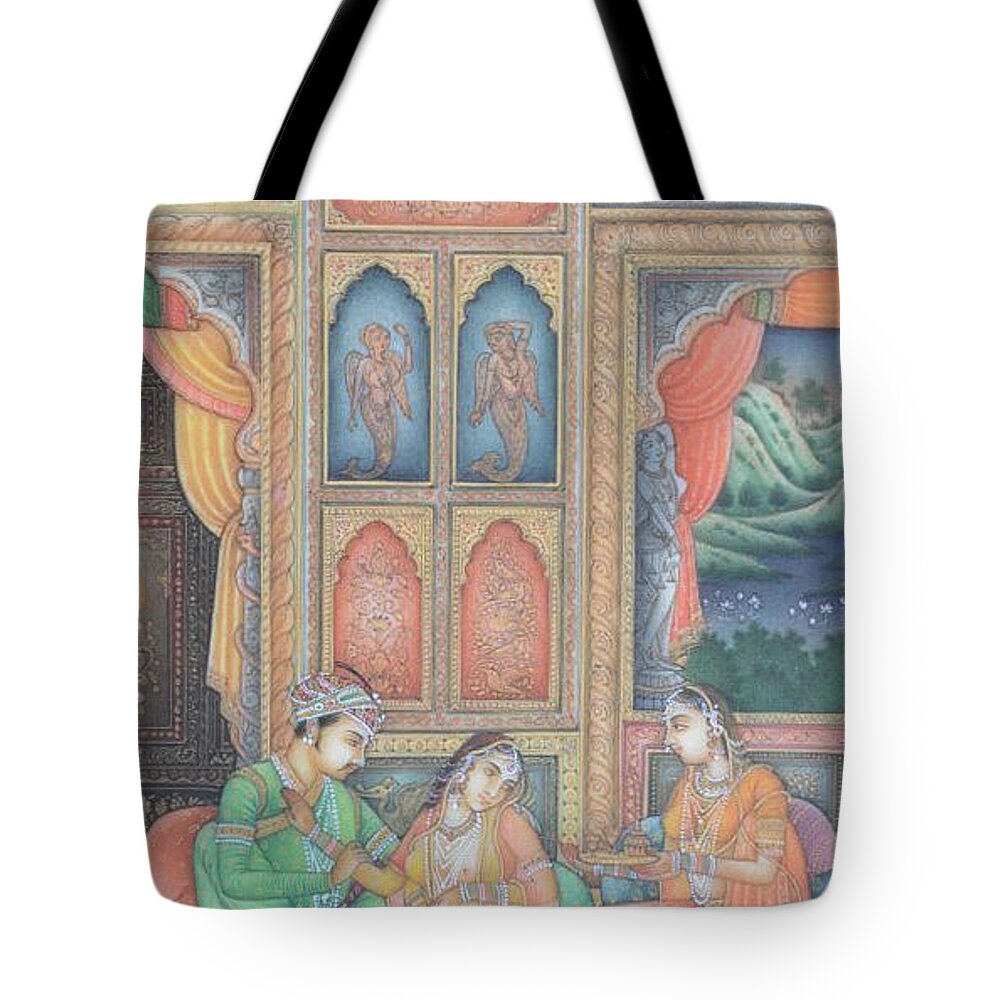This image features a detailed canvas tote bag with a black handle that extends out of the frame against a white background. The bag showcases a vibrant, intricate artwork depicting an Indian scene. The central focus is on three figures; a man and two women, adorned in opulent traditional Indian attire characterized by rich colors, elaborate jewelry, and headdresses. 

The man, dressed in lavish gold and green, is seated and holds the arm of a woman in yellow and red, who wears long necklaces and a similar headdress. Another woman in the scene, dressed in an orange traditional outfit laden with jewelry, appears to be offering something, likely a beverage or food, on a tray. Their skin tones are rendered in a faint yellow, adding to the exotic and historical feel of the scene.

The backdrop of the artwork is equally elaborate, featuring a doorway with a colorful curtain in blue, maroon, and yellow on the left, and a window with a view of trees and shrubs on the right, both adorned with similarly patterned drapery. Above the figures, the scene extends to include stained glass windows; the top ones are blue with angelic figures, while the bottom ones are maroon, displaying abstract designs in different shades of white and brown. The setting appears to be a luxurious interior, possibly a palace, given the intricate details of the background objects like mermaid art on the walls, large statues of women, and gold-plated photo frames.